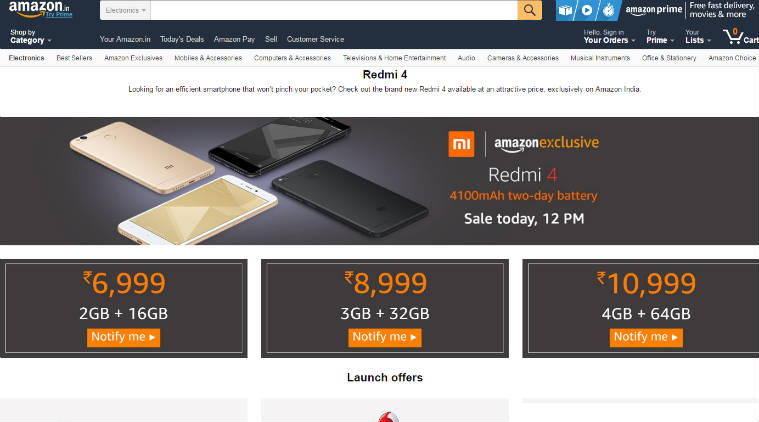The image is a screenshot of the Amazon.in app interface, displaying its online store layout. The header is colored dark blue and features multiple tabs which include "Shop by Category," "Your Amazon.in," "Today's Deals," "Amazon Pay," "Sell," "Customer Service," "Hello, Sign In," "Your Orders," "Prime," "Your Lists," and "Cart." There are also notifications regarding "Free Fast Delivery Movies and More with Amazon Prime," and a search bar situated at the top.

The central white background area of the interface is populated by various navigation tabs such as "Electronics," "Best Sellers," "Amazon Exclusives," "Mobiles & Accessories," "Computers & Accessories," "Televisions," "Home Entertainment," "Carriers," "Cameras & Accessories," "Music & Instruments," "Office & Stationery," and "Amazon Choice."

Below the navigation tabs, there's prominently displayed promotional text and an image for the "Redmi 4" smartphone. The promotional text reads: 
"Looking for an efficient smartphone that won't pinch your pocket? Check out the brand new Redmi 4 available at an attractive price, exclusively on Amazon."

The center of the image showcases three Redmi 4 phones – two in black and one in gold – set against a black background. Text on the right side of the image, written in white and yellow, states:
"Amazon Exclusive Redmi 4 with 4100mAh Battery, Two-Day Battery, Sale Today 12 PM."

An orange and white Redmi logo is also present. At the bottom of the image, pricing details are provided in orange text, alongside the specifications in white text. The available options and corresponding prices are:
- 2GB RAM + 16GB Storage for 6,999 INR (with a “Notify Me” button)
- 3GB RAM + 32GB Storage for 8,999 INR
- 4GB RAM + 64GB Storage for 10,999 INR